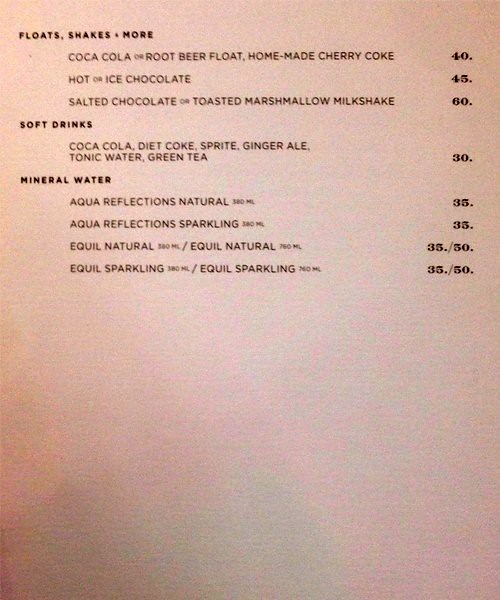The image captures a vintage restaurant menu, slightly discolored with time, giving it a pinkish hue. The menu is set against a cream-colored background. At the top left, in bold black capital letters, it reads "FLOATS, SHAKES, AND MORE." Below that, the menu features a variety of offerings with prices following in bold. 

It starts with "Coca-Cola or Root Beer Float" and "Homemade Cherry Coke" priced at $0.40. Next are drink options like "Hot or Iced Chocolate" for $0.45 and the "Salted Chocolate Toasted Marshmallow Milkshake" for $0.60. 

Under the "SOFT DRINKS" category, listed drinks include Coca-Cola, Diet Coke, Sprite, ginger ale, tonic water, and green tea, each priced at $0.30. Additionally, the menu offers "Mineral Water" options, including "Aqua Reflections Natural" and "Aqua Reflections Sparkling" for $0.35, as well as "Equal Natural" and "Equal Sparkling" available at either $0.35 or $0.50.